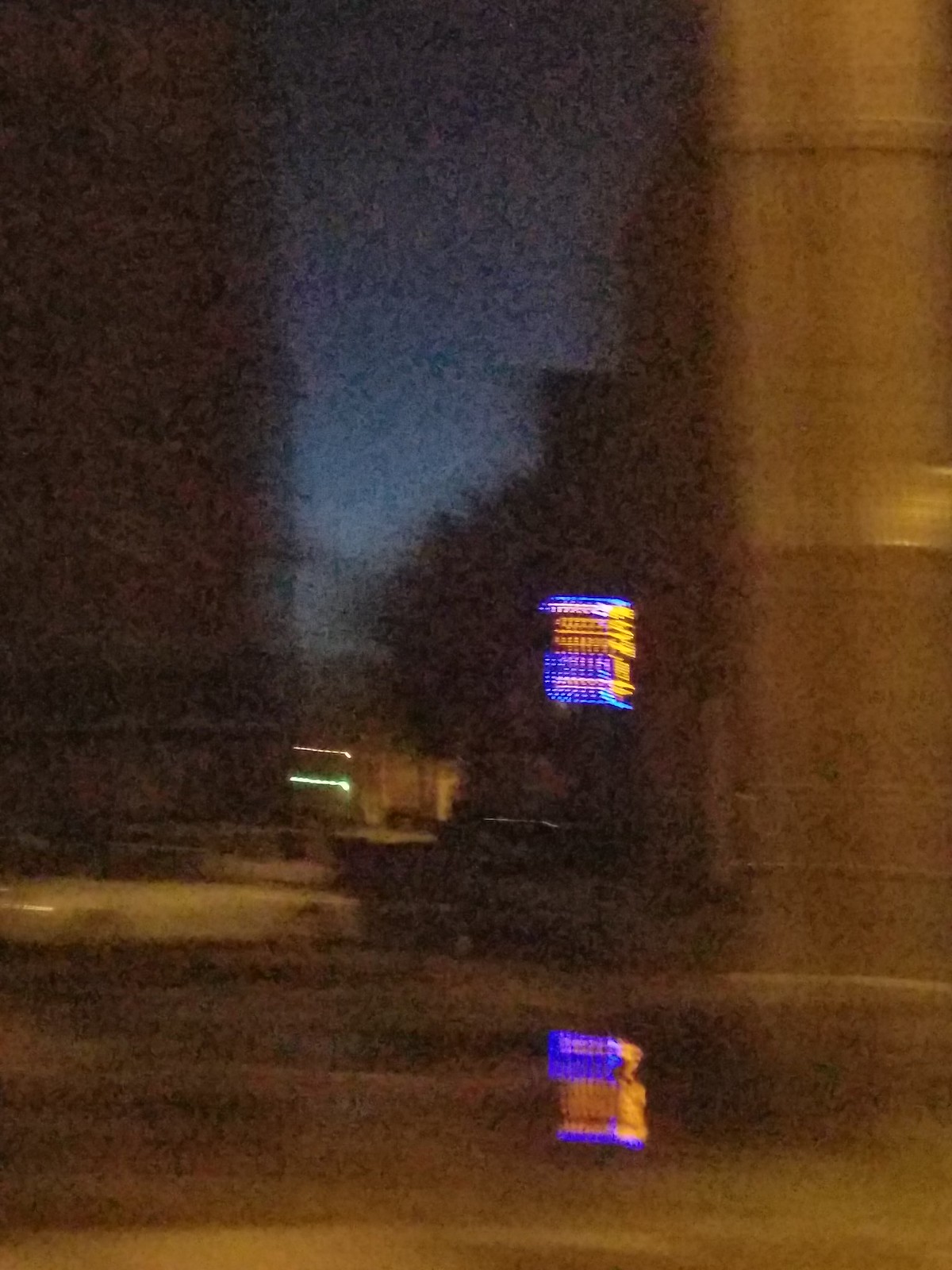The photograph, taken at night, presents a surreal and distorted scene resembling a digital glitch. In the center, a blurry white car is faintly visible, seemingly parked in front of a house which is partially obscured. The house itself is indistinct but suggested by the blurred lights and shadowy outlines. To the side, a dark silhouette of a tree punctuates the scene, adding an element of natural mystery. Above, the night sky transitions to a deep blue hue, occupying the top central portion of the image. A striking visual anomaly dominates the picture: an overlapping array of blue, orange, and yellow lights that bend and reflect in a glitch-like manner, creating an otherworldly effect. These distorted lights seem to cascade and merge in an unnatural, almost symbiotic fashion, further adding to the enigmatic atmosphere of the photograph.